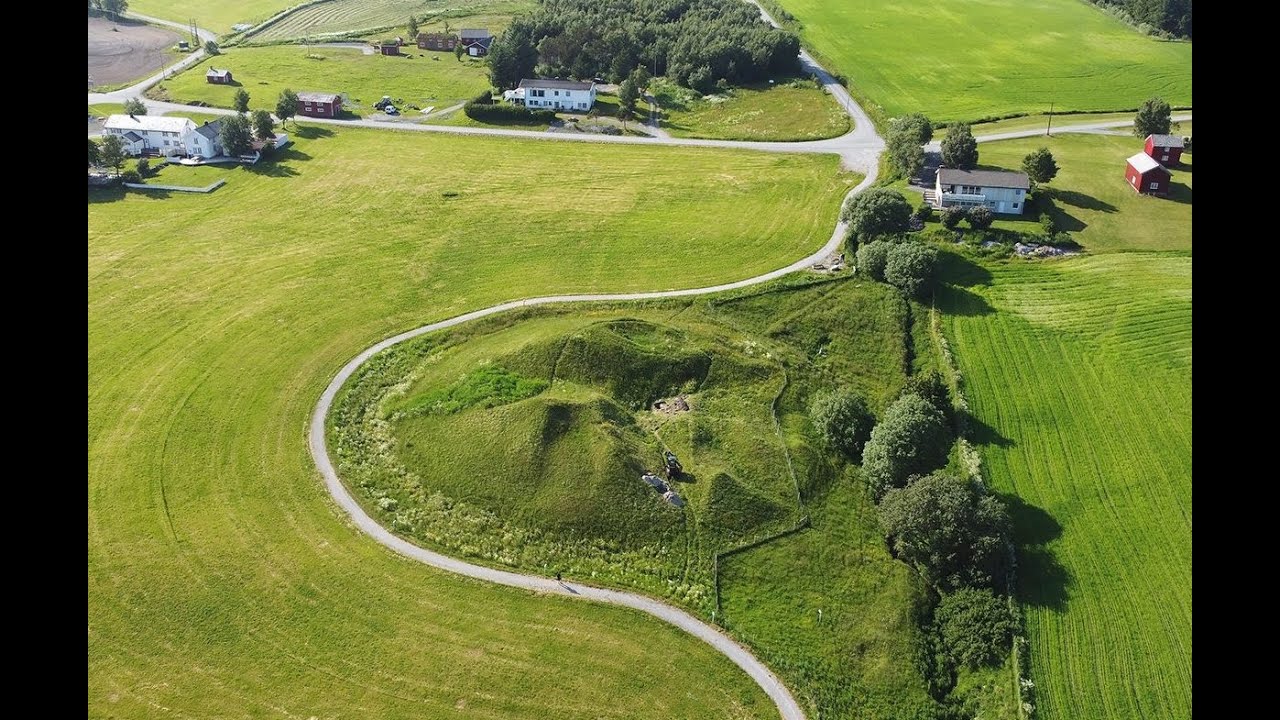An overhead aerial shot captures a sprawling rural landscape characterized by a large green field with varying shades and textures of grass. A winding gray path weaves through the scene, segmenting the area into distinct sections. Dotted sporadically across the field are several buildings, predominantly white with sloping roofs, standing two stories tall. On the top left corner, a white two-story house with a driveway sits adjacent to a small grove of trees. Various other structures, likely outhouses, are sparsely spread in the backdrop.

In the center of the image is a prominent green mound, surrounded by trees. The trees are arranged in a vertical line to the mound's right. In the top right corner, two red barns stand out, one with a white roof and the other with a gray roof. Close to these barns, on their left side, another white two-story house with a gray roof can be seen. The overall view is from a top-down perspective, making the buildings and landscape features appear smaller. Additionally, people can be seen walking along the intersecting roads, contributing to the tranquil, rural atmosphere of this outdoor setting.